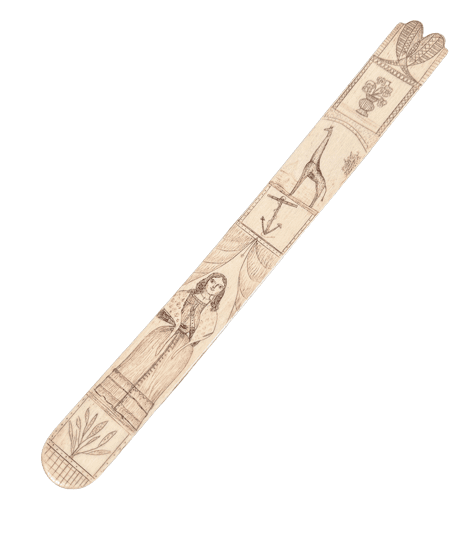The image showcases a long, flat, light brown wooden stick, reminiscent of a Popsicle stick, with a series of detailed carvings along its surface. At the top, there are two small, rounded designs resembling tiny wings or half circles set side by side. Directly below these designs is a sketched vase, framed to give a painting-like effect, with a bouquet of flowers inside. Continuing down the stick, there is an illustration of a giraffe viewed from the left side, next to a small tree. Below the giraffe, a carved boat anchor is enclosed within a rectangular border. Moving further down, there is an open curtain with a woman positioned underneath. The woman is dressed in a robe or shawl that conceals her feet and hands, which are behind her back. Finally, at the very bottom of the stick, there is a small plant situated beneath the figure of the woman. The entire series of designs runs diagonally from the top right to the bottom left of the stick, with the background kept white to highlight the intricate carvings.